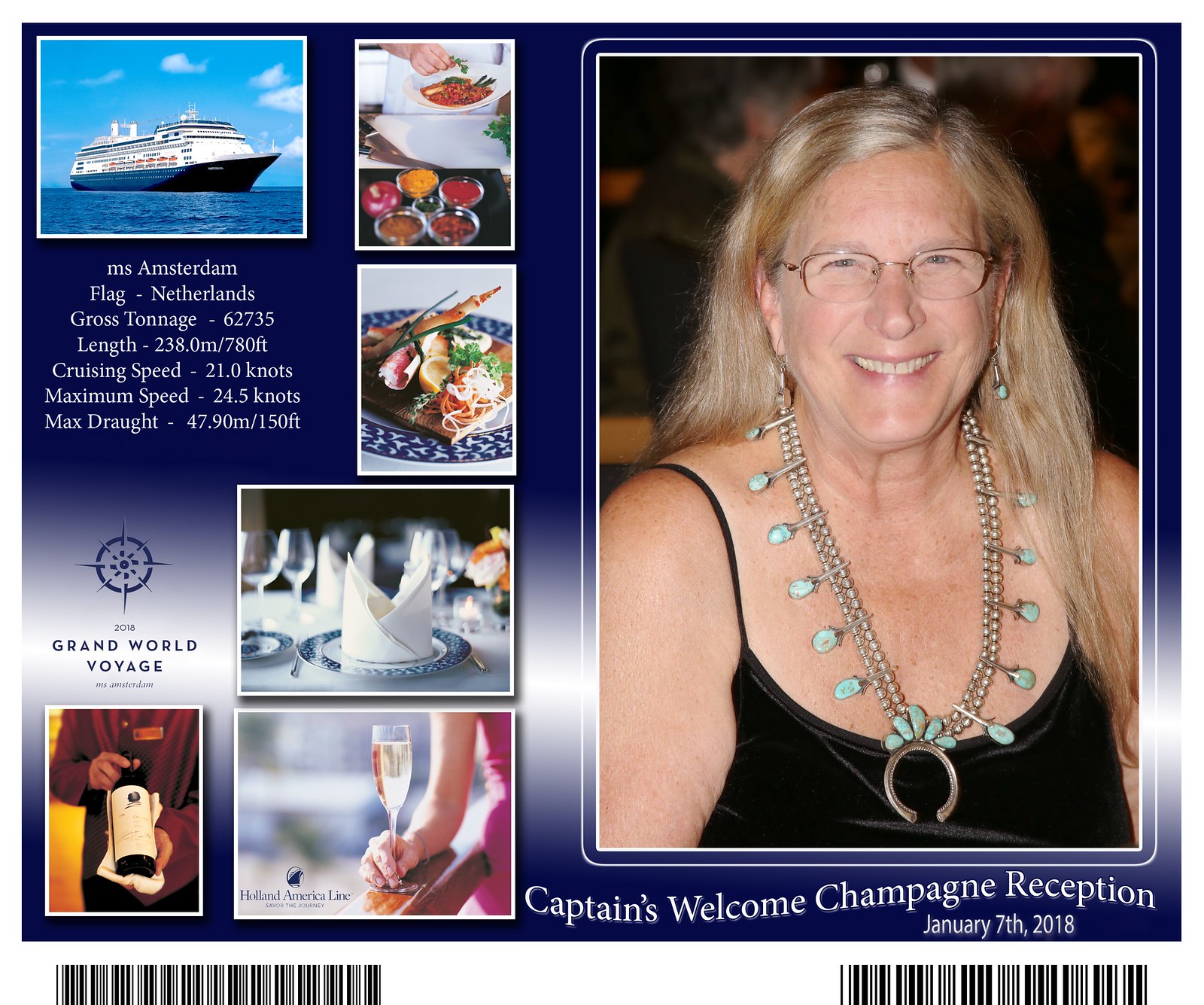This promotional brochure for the Captain's Welcome Champagne Reception on January 7th, 2018, highlights a luxurious experience aboard the MS Amsterdam during the Grand World Voyage. The centerpiece of the brochure features a smiling Caucasian woman in her 50s or 60s wearing elegant jewelry, including a distinctive horseshoe-shaped necklace adorned with blue jewels and two rows of beaded pearls. She is dressed in a black top with small straps and glasses. Surrounding her photo are smaller images: one of the cruise ship itself against a blue sky labeled with technical details like its flag and tonnage; another of a waiter presenting a bottle of champagne; a woman holding a glass of champagne; a set dining table; and several photos of the exquisite food offered on the cruise, including vegetables and lobster. The brochure also includes practical information about the cruise such as directions, length, cruising speed, and maximum draft. QR codes located at the bottom corners suggest the need for scanning, possibly for identification purposes during the voyage.